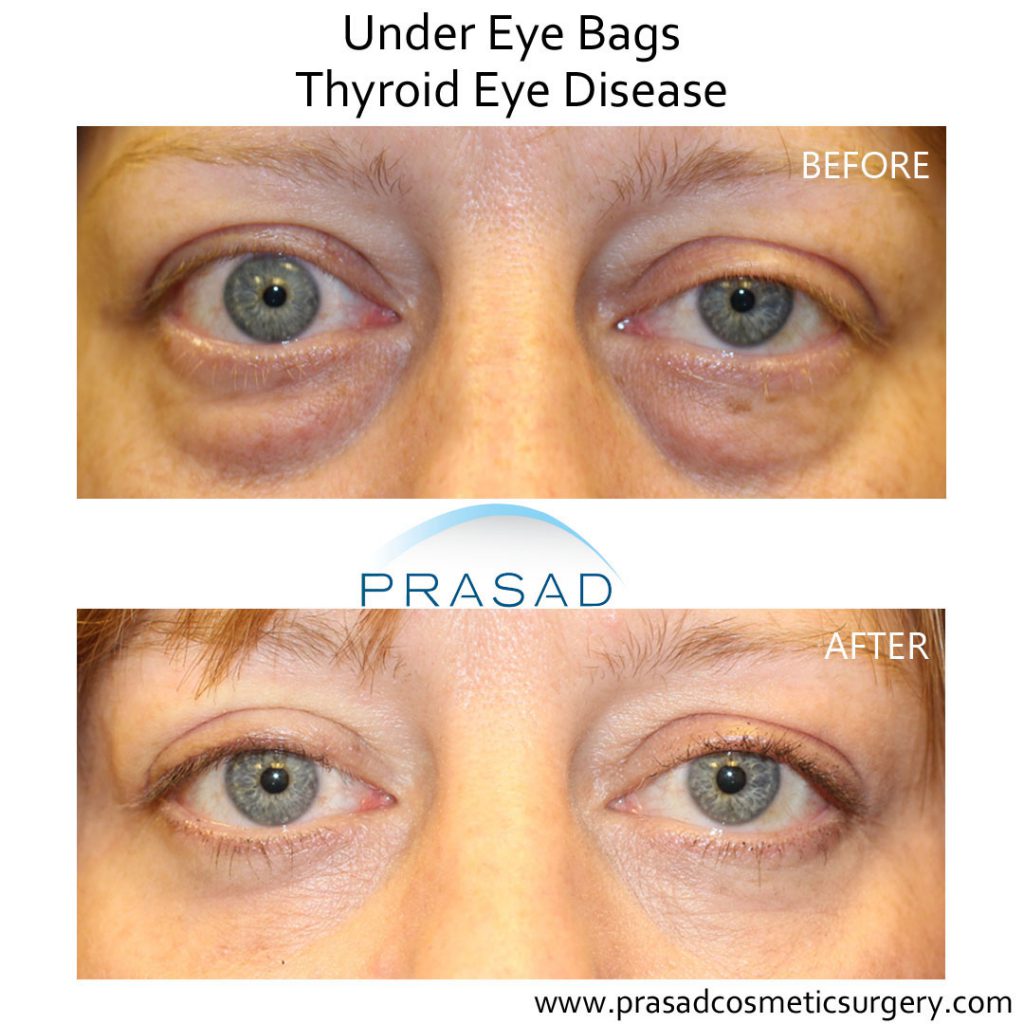The image features a before-and-after comparison of a woman’s eyes, showcasing the effects of a cosmetic surgery performed to address under-eye bags related to thyroid eye disease. The top section presents a photograph marked "BEFORE" in the upper right corner, depicting swollen under-eye bags with light brown spots, and red, irritated skin. The woman has light brown eyebrows and striking blue eyes. Above this image, the text reads "UNDER EYE BAGS THYROID EYE DISEASE." In contrast, the bottom section shows the same woman's eyes in a photograph labeled "AFTER" in the upper right corner. Here, the under-eye area appears tight, smooth, and free of discoloration and puffiness. Between the two images, the name "Prasad" appears in blue, set against a white background. The clinic's website, www.PrasadCosmeticSurgery.com, is prominently displayed at the bottom right corner of the image.